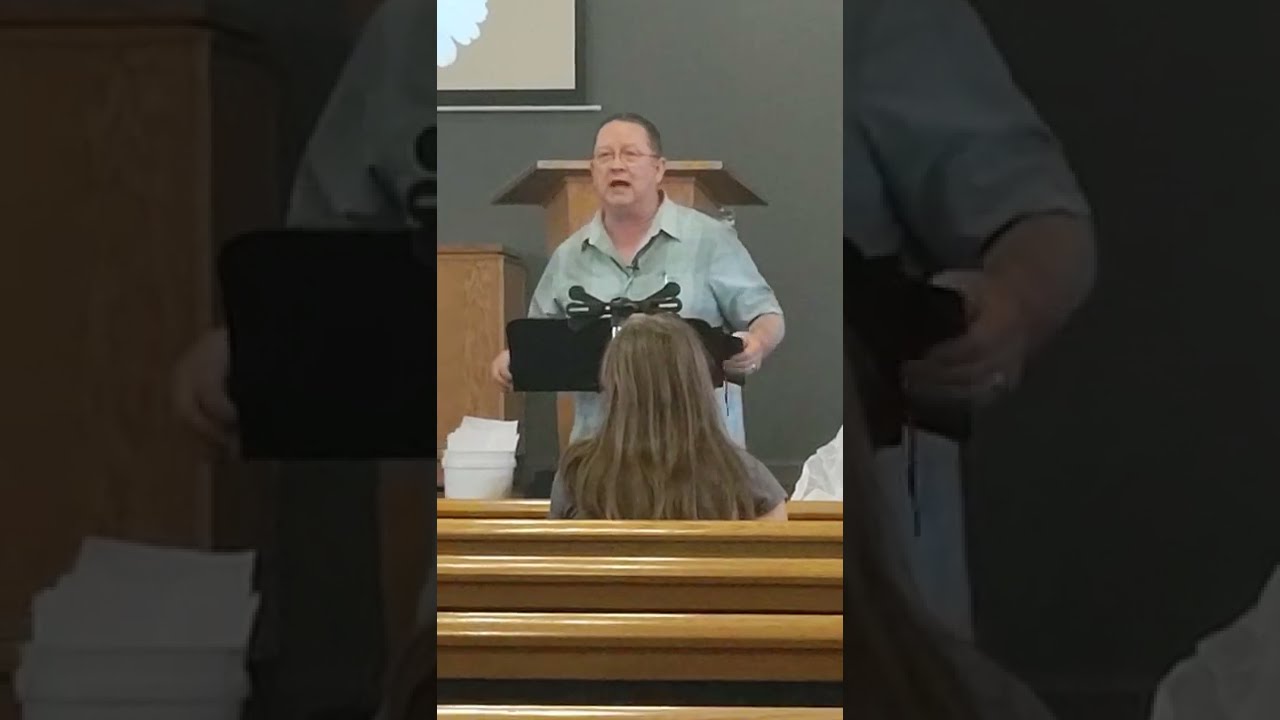In a serene and tidy church setting, a man, likely a pastor or priest, stands at the center of the photo delivering a sermon. He wears glasses, a green collared polo shirt, and has short hair. His arms rest on a black podium, which features a microphone stand. Behind him, a large LED screen is mounted on a gray wall, with additional wooden podiums visible in the background. The image also captures a white bucket filled with papers placed behind him. The seating area consists of clean, well-maintained wooden booths, and within one of these sits a young girl with long hair, attentively listening to the sermon. A fragmentary view of another person’s shoulder is visible, indicating a sparse but present audience. The overall ambiance is orderly and reflective, highlighting the pastor deeply engrossed in his preaching.